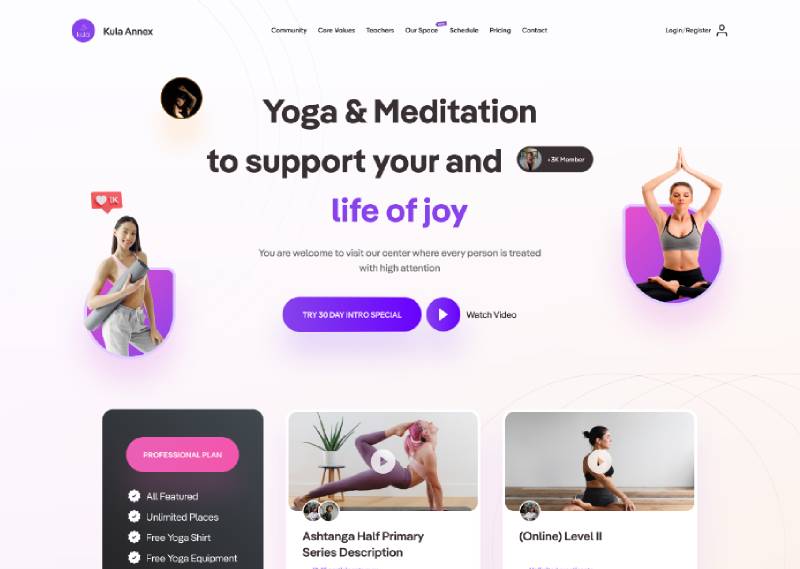Homepage of Kula Annex Yoga and Meditation Center

The homepage of Kula Annex features a welcoming and vibrant layout designed to promote their yoga and meditation services aimed at fostering a joyful life. Prominently displayed in bold black text at the center of the page is the tagline, "Yoga and meditation to support your life of joy," with the words "life of joy" highlighted in purple.

In the upper left corner, a purple circle with black text beside it reads "Kula Annex," positioned towards the center. The top navigation menu, displayed in black text, includes the following options: Community, Care Workers, Teachers, Our Space, Schedule, Pricing, and Contact. At the far right of the menu, there are options to "Login" or "Register."

Underneath the navigation menu, the page features a central image of a Caucasian woman in a yoga pose, seated in a crisscross position against a purple background. She is wearing a gray sports bra and black leggings. To the far left of the image, an Asian woman with light brown skin and black hair is depicted. She is dressed in gray pants and a gray sports bra, carrying a gray yoga mat.

Between these two figures, there's a welcome message: "You are welcome to visit our center where every person is treated with high attention." Below this message, a long purple oval button invites visitors to "Try 30-day intro special" in white text, accompanied by a circle with a white triangle pointing to the right, indicating a video to watch. Below the call-to-action, the homepage showcases two featured video thumbnails.

This homepage is designed to be both inviting and informative, encouraging visitors to explore the various offerings of the Kula Annex Yoga and Meditation Center.